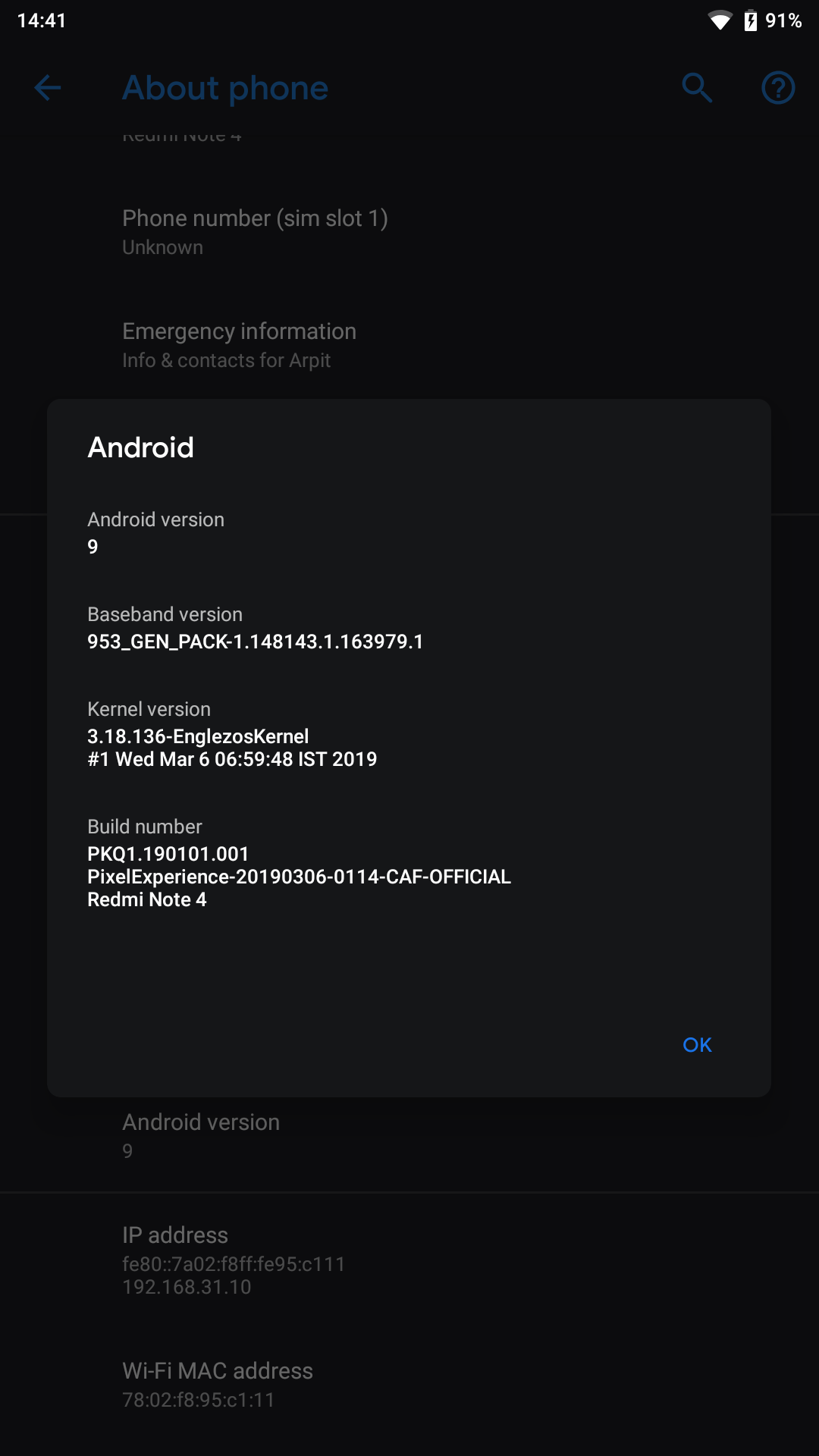The image shows a cell phone settings screen against a black background. In the upper left corner, the time is displayed as "14:41". In the upper right corner, the battery status is indicated at "91%", with a charging icon next to it, and a three-quarters full Wi-Fi icon.

Beneath this status bar, the main screen header reads "About Phone", accompanied by a search bar and a Help button. The top section of the settings lists critical device information: "Phone Number: Unknown", "SIMSWAT1", and "Emergency Information", which includes "Information and Contacts for RPIT".

Further down, the screen reveals the cell phone's detailed technical details. It lists "Android version: 9" along with the device's "IP address: FE80:FA02:F8FF:FE95:C111 / 192.168.31.10" and "Wi-Fi MAC address: 78:02:F8:95:C1:11".

A pop-up on the screen provides additional system specifics:
- "Android version: 9"
- "Baseband version: 953_GEN_PACK-1.148143.1.163979.1"
- "Kernel version: 3.18.136 (Goslios) #1 Wed Mar 6 2019, 06:59:48 IST"
- "Build number: PKQ1.190101.001"
- "Pixel Experience version: 20190306-0114-CAF-official"

The screenshot encapsulates a comprehensive summary of the device specifications and system information in a very concise yet detailed manner.